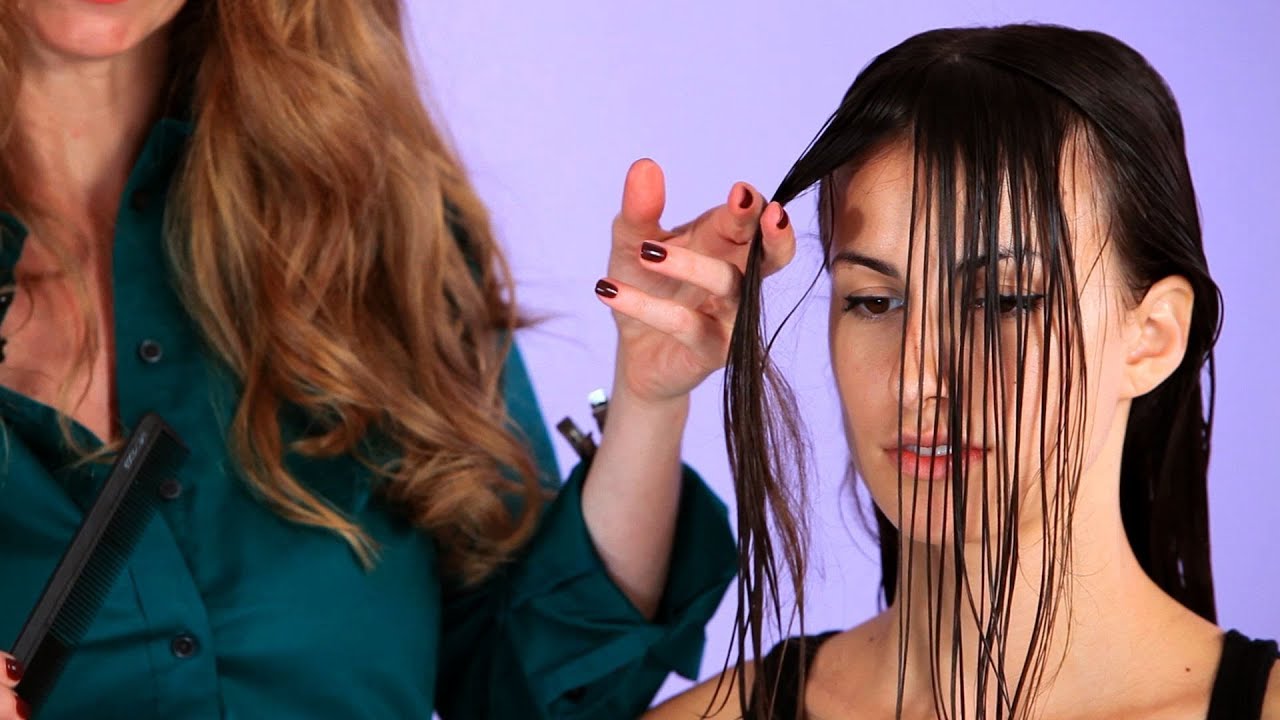In this image, we see a Caucasian woman seated and getting her hair styled, looking down solemnly at the floor. Her dark black hair is sectioned into bunches, with stray strands hanging down in front of her face. The stylist, whose face is partially out of frame, is visible from her chest to her chin on the left side of the image. She is wearing a buttoned-up, dark green shirt and has brown hair. The stylist is holding the customer's hair with her left hand while holding a black comb in her right hand. Her nails are painted a reddish-purplish wine color. The background of the image features a lavender hue, adding a subtle contrast to the scene.